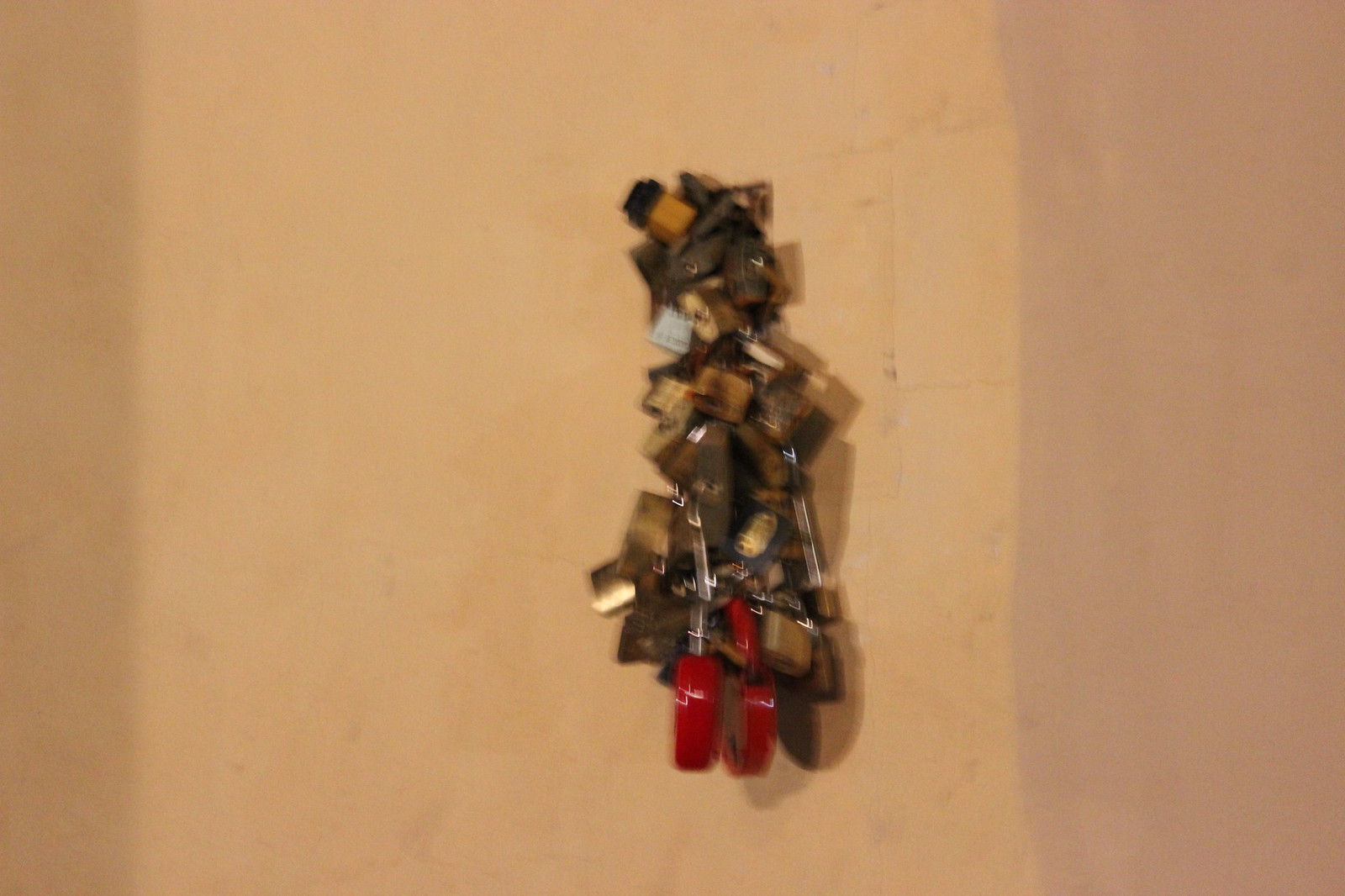The image features a background of a medium tan tone. On the eastern and western edges, there are strips of a darker tan, with the strip on the right being thicker. At the center is a heap of small metal pieces resembling padlocks or lockets in various shapes and sizes, stacked vertically from north to south. The heap features predominantly gold- and silver-toned locks, interspersed with a few dark gray or black ones. Notably, at the bottom of the image, there are two large, shiny red locks. The locks appear to be interconnected, forming a vertical blob that occupies about two-thirds of the image's length. The background shows a plain beige wall, with shadows and scuffs, and on the right side, the wall takes on a slightly pink hue with visible dents and patches. The overall appearance of the metal heap and the partially covered ends, combined with repetition and various color tones, underscores the intricate and interwoven nature of the locks.